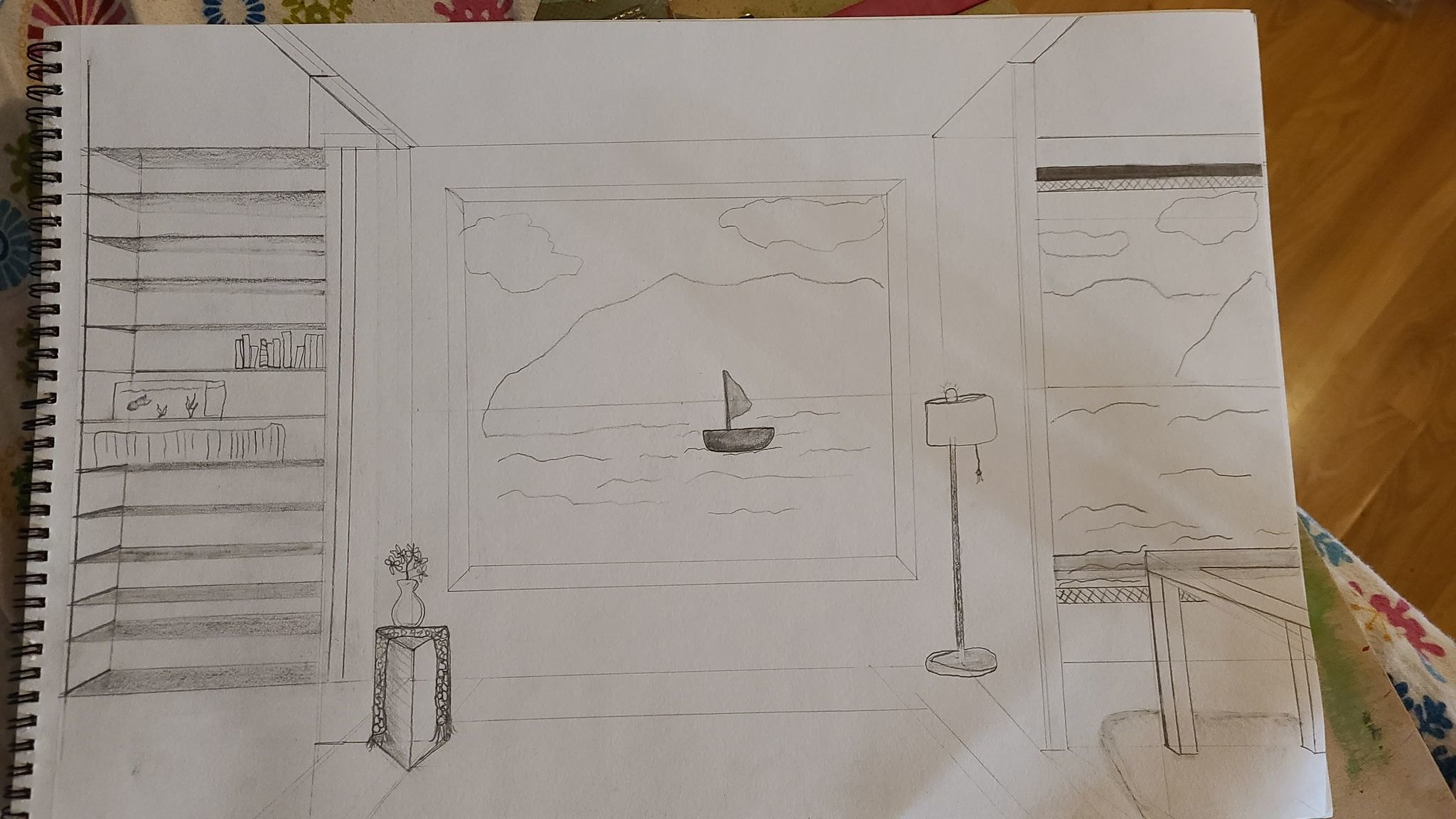This is a close-up photograph of a detailed pencil drawing on white sketchbook paper, secured with a black metal binder on the left side. The sketchbook rests on a multicolored floral tablecloth featuring yellow, blue, red, and green flowers, partially visible against a light brown laminate floor with signs of water damage. In the drawing, a living area is depicted with a bookcase on the left, housing a few books and a fish tank with a couple of fish and some aquatic plants. Next to the fish tank is an object that resembles a ruler. A vase with flowers sits on a triangular, dark grey stand with embroidery. To the right, a tall floor lamp with a cylindrical lampshade and a round pedestal base illuminates the scene. The focal point of the drawing is a window view of an ocean, where a sailboat with a triangular flag is sailing beneath a cloudy sky, with mountains faintly sketched in the background. Also sketched are smaller details like a floor grate, a railing-like structure, and an additional picture frame depicting similar mountainous and aquatic scenery, all adding to the intricate composition of the room.